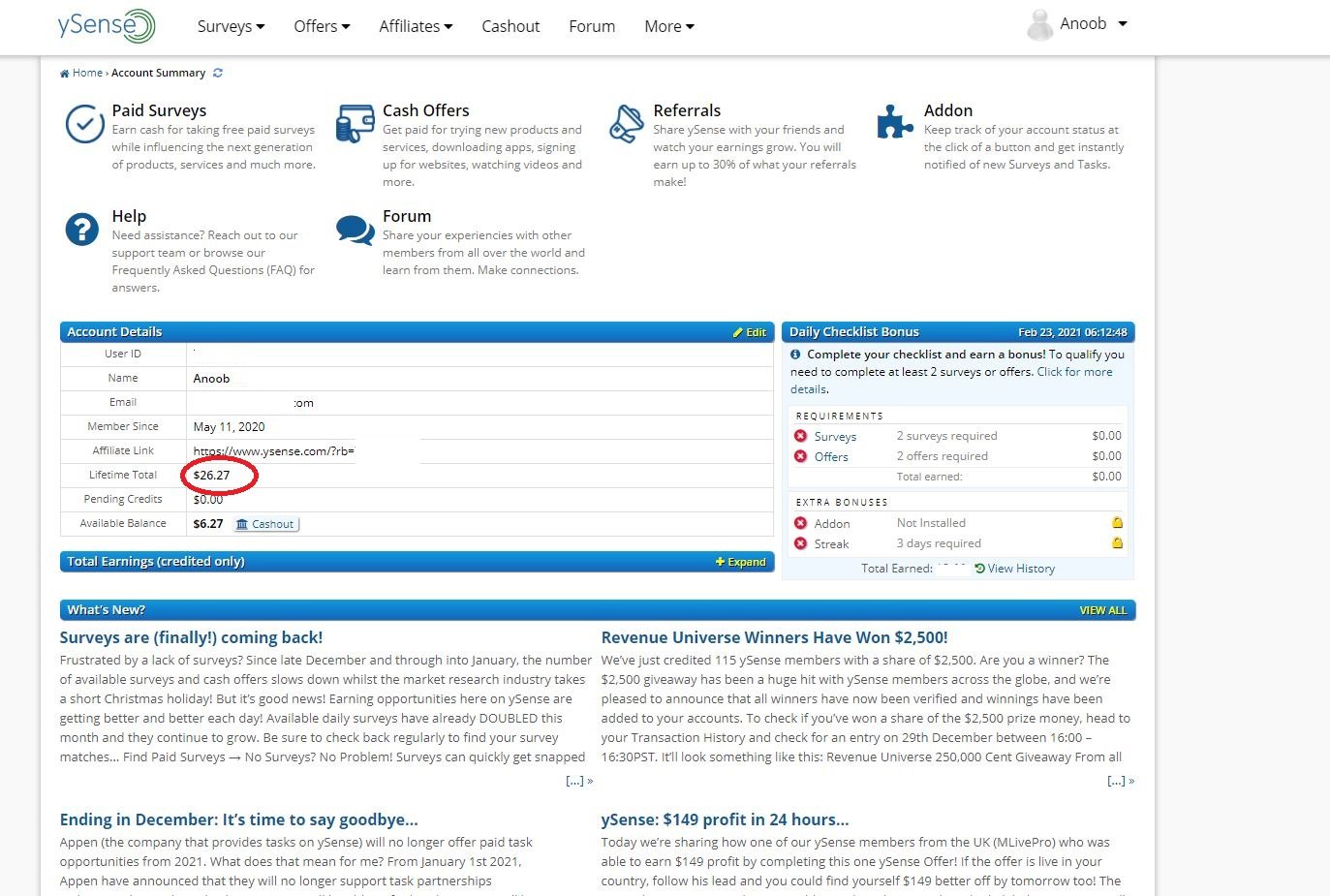This landscape-oriented screenshot features the dashboard of a YSense user account. The screen is presented with a light gray background on the left and right sides, while the rest of the background is white. At the top, a navigation bar runs across the screen starting with the YSense logo, followed by the navigation options: Surveys, Offers, Affiliates, Cashout, Forum, and More. In the upper right-hand corner, the username "aNooB" is displayed.

Below the navigation bar, the screen is divided into multiple sections. The first row on the left lists home navigation options: ‘Home,’ 'Account Summary,’ and a refresh icon button. The subsequent menu options are organized in a grid, detailing 'Paid Surveys,' 'Cash Offers,' 'Referrals,' 'Add-on,' 'Help,' and 'Forum.'

The main content area is organized into two columns. The left column includes an 'Account Details' section, highlighted in blue. Underneath, there is detailed account information displayed in white:
- User ID: name
- Username: aNooB
- Email
- Member since: May 11, 2020
- Affiliate link 
- Lifetime total earnings: $26.27
- Pending credits 
- Available balance: $6.27

The right column features a 'Daily Checklist Bonus' for February 23rd, 2021, which details the requirements to earn a daily bonus. To qualify, users need to complete at least two surveys or offers. The checklist is broken down as follows:
- Surveys: two surveys required
- Offers: two offers required
- Add-on: not installed
- Streak: three days required

The bottom of the right column provides updates with a 'What's New?' section, featuring announcements such as "Surveys are finally coming back," "Revenue Universe ending in December," and "YSense: $149 profit in 24 hours."

This descriptive caption provides a comprehensive overview of the YSense dashboard and the user's account summary as portrayed in the screenshot.